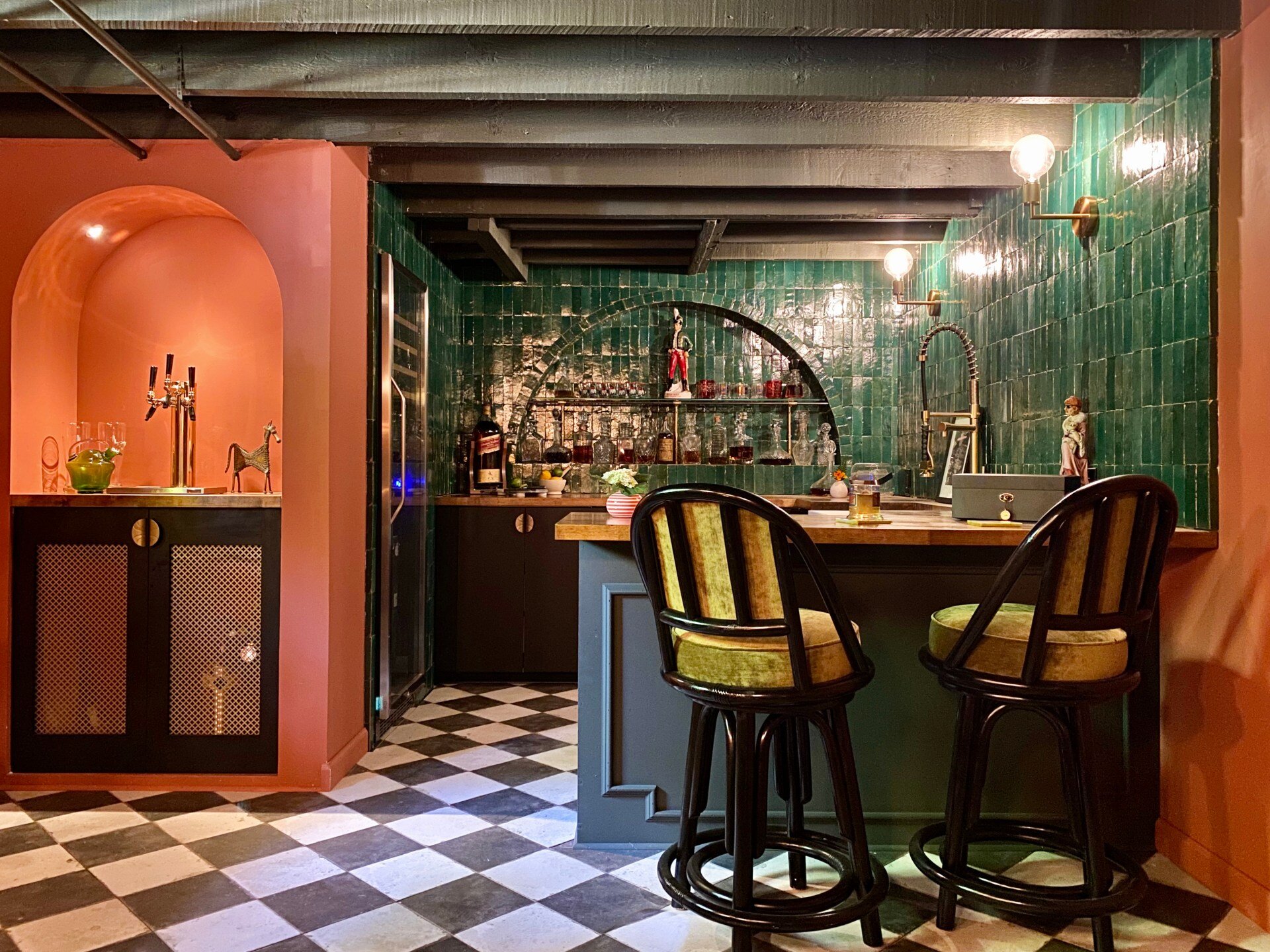This detailed photograph captures a vibrant and eclectic kitchen area. The centerpiece is a blue countertop with a light wooden top that wraps around and extends into a bar on the right side, fronted by two yellow stools with metal circular frames. A stainless steel fridge stands to the left, accompanied by green rectangular vertical tiles on the backsplash. The floor features a striking black-and-white checkered pattern. 

To the left, there's an inset archway in the pinkish-orange wall, housing a sink, tap, and small figures, including a horse. The archway also features a shrine-like setup with a small greenish-yellow bottle and two cups. The kitchen is decorated with various items, such as a pink and white striped pot with white flowers, a partly drunk beer, and a metallic cash box with gold detailing. 

On the bar area’s right side, shelves display an array of drinks, complemented by a whimsical small Elvis statue at the top. Ambient lighting highlights the eclectic decor, enhancing the kitchen's unique charm.